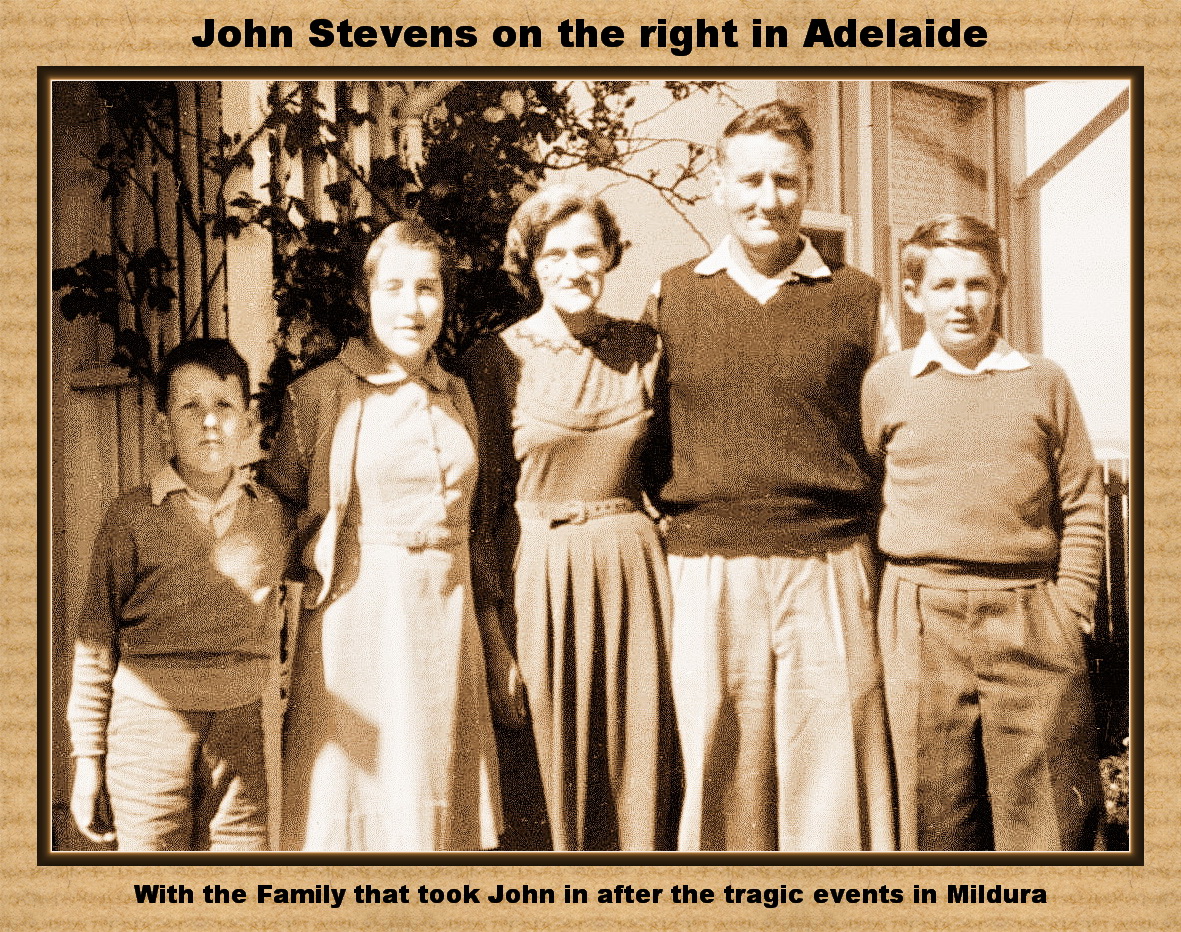This is an old sepia-toned photograph framed with a textured cardboard-like brown border and a thinner dark brown inner border. The image captions read "John Stevens on the right in Adelaide" at the top and "with the family that took John in after the tragic events in Mildura" at the bottom. Five figures pose outdoors in front of some plants or trees: on the far left is a young boy wearing a sweater, next to him stands a woman in a dress and cardigan, the central figures include another man and woman, and on the far right is John Stevens, a young man in a cardigan sweater and pleated pants, with the family who cared for him following the unfortunate events in Mildura. The photograph, characterized by its brown and lighter shades, exudes a sense of nostalgia and history.